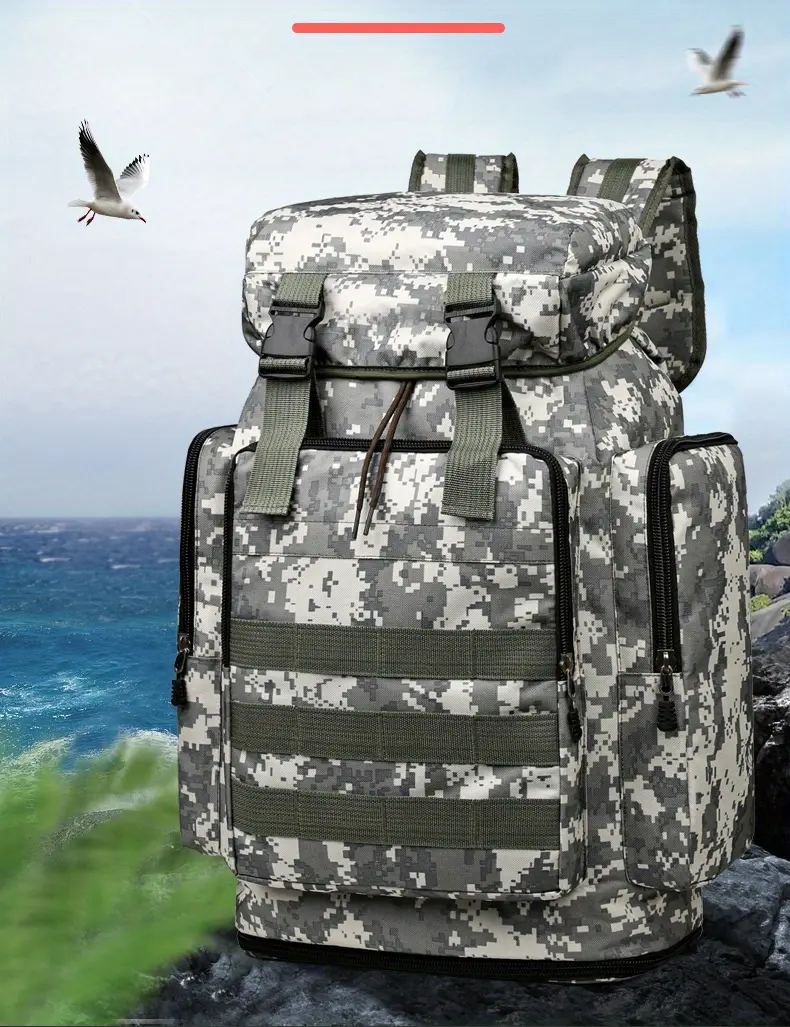In the foreground of this rectangular image, a camouflage backpack with military-style green and gray fabric rests prominently on a gray rock. The backpack features multiple details, including black clips for closures, green elastic straps and cords for adjustments, side pouches with black zippers, and a main zipper on the back. It has green straps on the front and brown drawstrings peeking from the top flap. Surrounding the rock, specks of greenery are visible, particularly on the left and behind the backpack.

In the background, the scenery captures an expansive ocean under a partly cloudy sky with patches of blue visible. To the right, a rugged sea cliff adds to the coastal landscape. Two seagulls are seen flying—one on the left and one on the right. An orange, oval-shaped thin line is noticeable in the sky near the top center of the image. The daylight and composition of the scene emphasize the serene yet detailed outdoor setting.